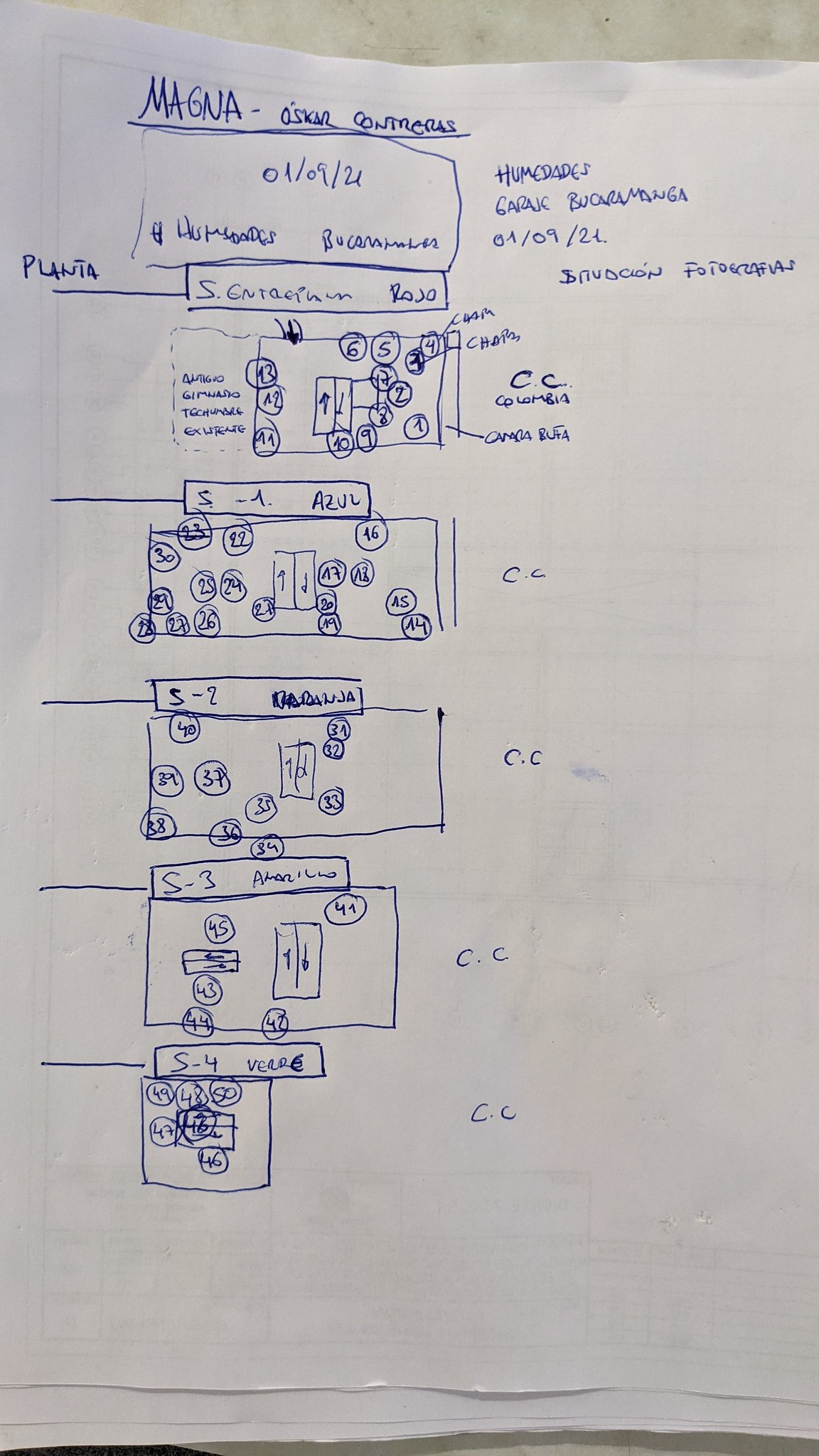The image depicts a multi-layered white sheet of paper, although the top layer is the only one clearly visible. On the translucent reverse side, faint impressions of diagrams and graphs emerge, though their specifics remain indistinct. The focal point is the handwritten content covering the top layer, penned in blue ink, which outlines a structured plan or an organization scheme. 

The header of the document reads "Magna - Oscar Contreras," suggesting a Spanish origin. It bears a date, "01/09/21," accompanied by a few names, although the handwriting makes these names difficult to decipher. Directly beneath this header, within a rectangular box, several Spanish words appear, including "Rojo." To the left of this box, a line is inscribed with the word "Planta."

Below this section is a series of diagrams, each sequentially detailed with numbers and annotations:

1. The first diagram is a rectangle labeled with numbers 1 through 13.
2. Beneath it, another chart features numbers such as 30, 22, and 25.
3. This is followed by a third diagram identified by the label "S2," containing numbers 39, 40, and 32.
4. Further down is another diagram marked "53 Amarillo," showcasing numbers like 45, 43, 44, 42, and 41.
5. The final diagram is marked "5-4" and "Verde," presented in pink, with numbers 49, 44, and 50.

To the right of these detailed diagrams, the initials "CC" are prominently featured.